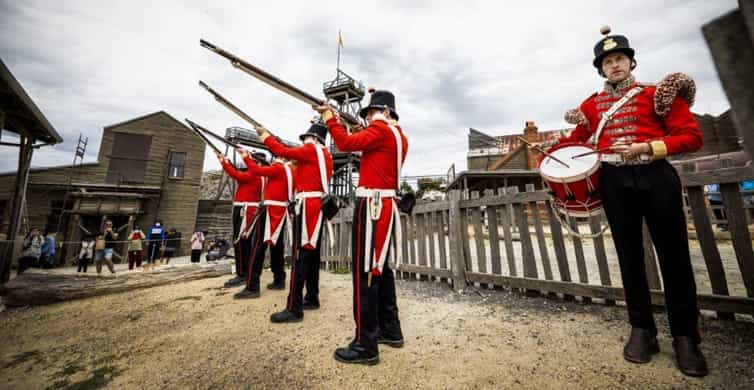In this photograph, five soldiers, dressed in red jackets with white suspenders and black slacks featuring red stripes down the sides, are depicted in a scene that appears to be a historical reenactment at a military fort. Four of these soldiers are centered in the foreground, raising their long-barreled muskets into the air as if firing a salute. To the right stands a fifth soldier, similarly attired, playing a drum and looking towards the camera. The background features a small brown wooden picket fence and wooden log structures, with tower-like elements hinting at the setting's historical significance. The sky above is overcast, adding a somber tone to the scene. Additionally, a group of onlookers, likely tourists, are visible to the left, observing the reenactment.